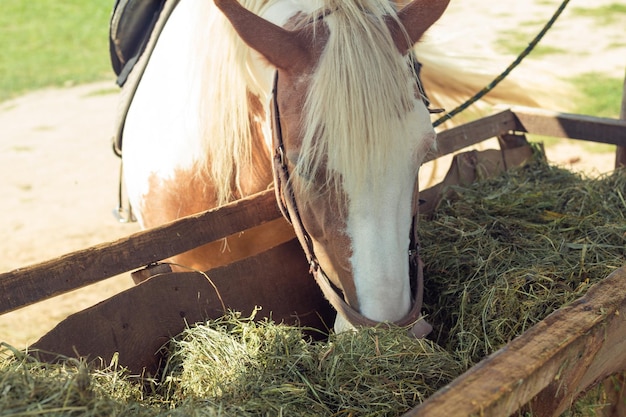The image captures a tan and white horse or pony with a light yellow mane, featuring a distinctive white flash down the center of its face and tan on its cheeks. The horse's ears are relaxed and its nose is buried in a bale of very green and fresh hay that stretches from the bottom left corner to the mid-right portion of the image. The animal is tied to something, indicated by a rope leading off the page, and appears to be equipped with a black saddle that is partially visible. In the background, there is a mix of green grass and brown dirt, suggesting a natural outdoor setting with the sun high in the sky. The horse's front end, including its shoulders and chest, displays a mix of tan and white coloration, and it is feeding from a rusty-looking wooden container filled with the greenish-yellow hay. Additionally, there are hints of a headstall around its face.